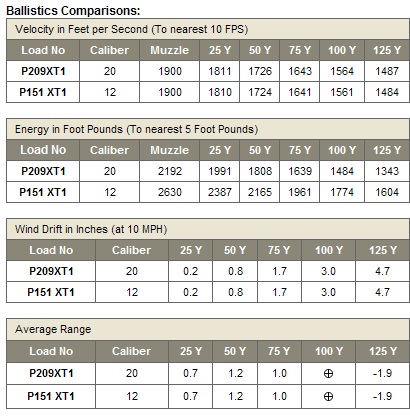This detailed photograph captures a comprehensive ballistics comparison chart, subdivided into four distinct sections. At the top, the chart is titled "Ballistics Comparisons." The sections are methodically labeled from top to bottom: Velocity (measured in feet per second to the nearest 10 FPS), Energy (in foot-pounds to the nearest five foot-pounds), Wind Drift (in inches at 10 miles per hour), and Average Range. Each section provides detailed categories, including Load Number, Caliber, Muzzle, and distance metrics at 25 yards, 50 yards, 75 yards, 100 yards, and 125 yards. Notably, the chart compares the same two load numbers, P209 XT1 and P151 XT1, across all categories, likely related to specific firearm or ammunition types. The visual presentation includes a tan bar, a darker brown bar, and two white bars containing various columns filled with text and names.